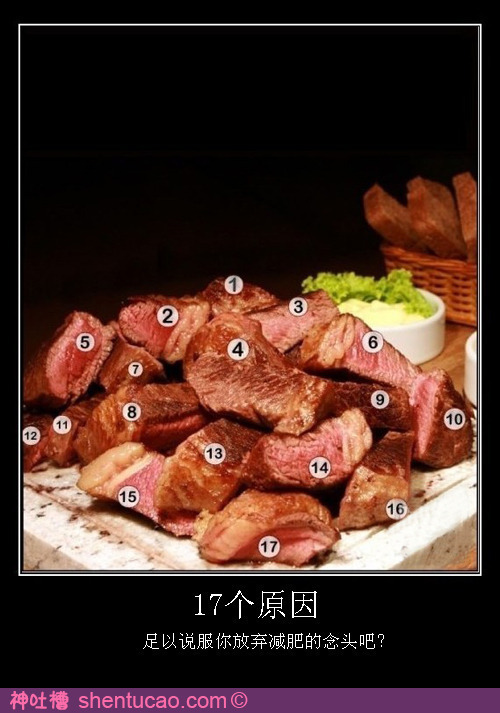This detailed, full-color photograph depicts a variety of cooked meat cuts, most likely beef or pork, served on a white ceramic platter. Each slice, which appears to weigh approximately two to three ounces, is marked with small white circles containing black numbers ranging from 1 to 17. However, the image lacks a legend to explain what these numbers signify. The meat appears medium rare, with shades of light brown, red, and pink, along with bits of beige fat showing some browning.

In the background, on the wooden countertop, there is a wicker basket containing three pieces of wheat bread, characterized by their brown crust and interior. Accompanying the basket is a round ceramic dish with dark green lettuce and some onions, adding a pop of color to the scene.

Surrounding the image is a larger black rectangle that features the numeral "17" in white, accompanied by Japanese text and a question mark. Below this, there is a small purple rectangle with additional Japanese text in pink and the URL "shentucao.com" along with a copyright symbol. Despite the elaborate presentation and various elements, the precise meaning of the numbered meat cuts remains unidentified due to the absence of a corresponding key.